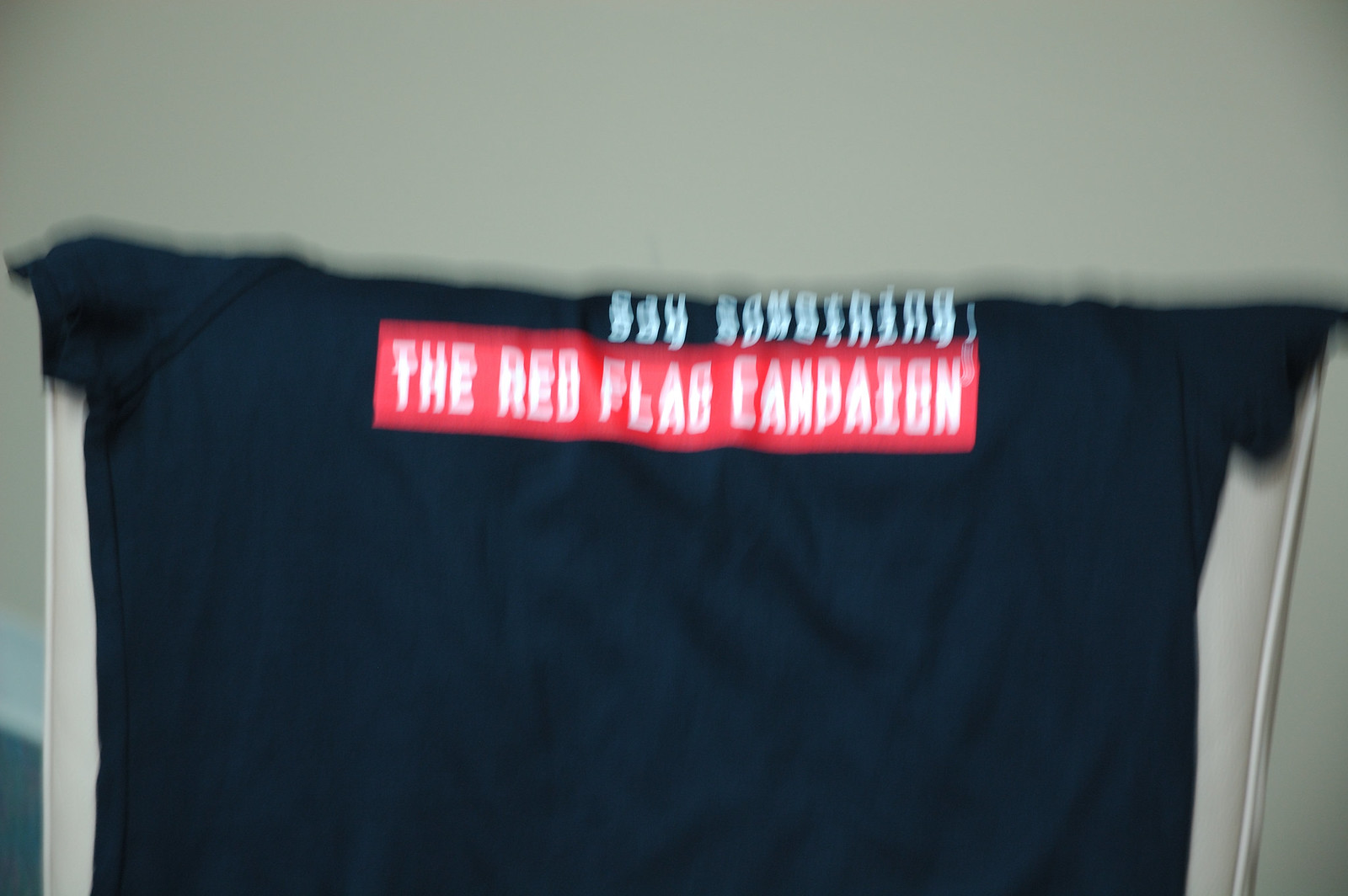This is a very blurry horizontal photograph of a navy blue t-shirt draped over the back of a tan upholstered chair, possibly made of wood. The image prominently displays the chest area of the t-shirt, as the collar and upper portion are out of view, folded over the chair. Blurred but visible, the t-shirt features the phrase "SAY SOMETHING" in white letters, positioned above a horizontal red rectangle. Inside the rectangle, also in white capital letters, it reads, "THE RED FLAG CAMPAIGN." The background consists of a beige wall, adding to the overall light color scheme framing the dark-toned t-shirt. The short sleeves of the t-shirt are partially visible, contributing to the perception of the shirt being casually draped.